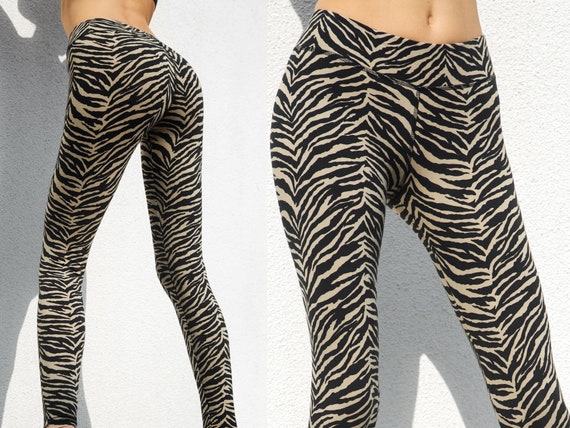The photograph portrays a woman wearing zebra-patterned leggings, shown from her belly button down to just above her ankles. The image is split into two angles: the first one captures her from behind, leaning against a white, stucco-textured wall with her shadow cast in front of her; the second angle shows her from the front, revealing her exposed belly button and a slight shadow above her. Both views highlight the distinct black and white zebra stripes of the tight-fitting leggings she wears, with careful attention to the lighting that accentuates her silhouette against the white background.